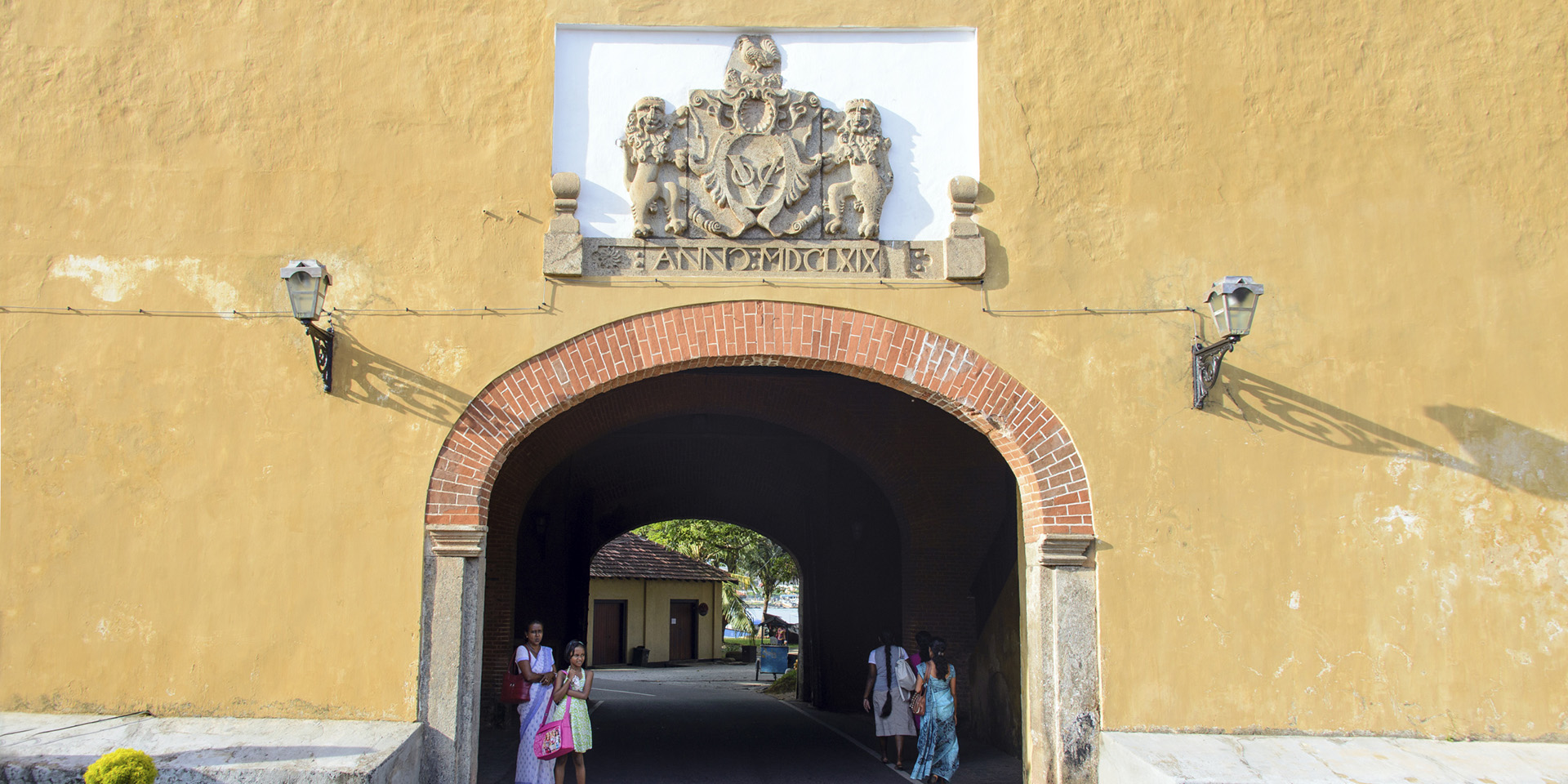The image depicts an archway entrance to a tunnel set in an old, weathered mustard yellow wall, with the paint noticeably chipping. Flanking the entrance are two metal light fixtures housing single bulbs. Above the archway, there is a stone sculpture resembling a coat of arms or a shield, possibly adorned with two creatures and partially legible inscriptions or symbols, such as the letters "MD."

Inside the tunnel, four women are visible. On the left side, one woman is a young girl in a yellow dress accompanied by a pink bag, while an older woman stands beside her, dressed in a white and blue dress and carrying a burgundy bag. On the right side, two women are walking away from the camera; one wears a cyan and dark blue dress with a brown bag, and the other has a long ponytail, dressed in a gray shirt and skirt, carrying a white bag.

The view extends through the tunnel, revealing a building with two brown doors, a roof likely covered with shingles, surrounded by green trees, and a glimpse of the sky. The architecture and attire suggest a setting possibly in India or another part of South Asia, with the women dressed in traditional saris, contributing to the cultural and historical ambiance of the scene.